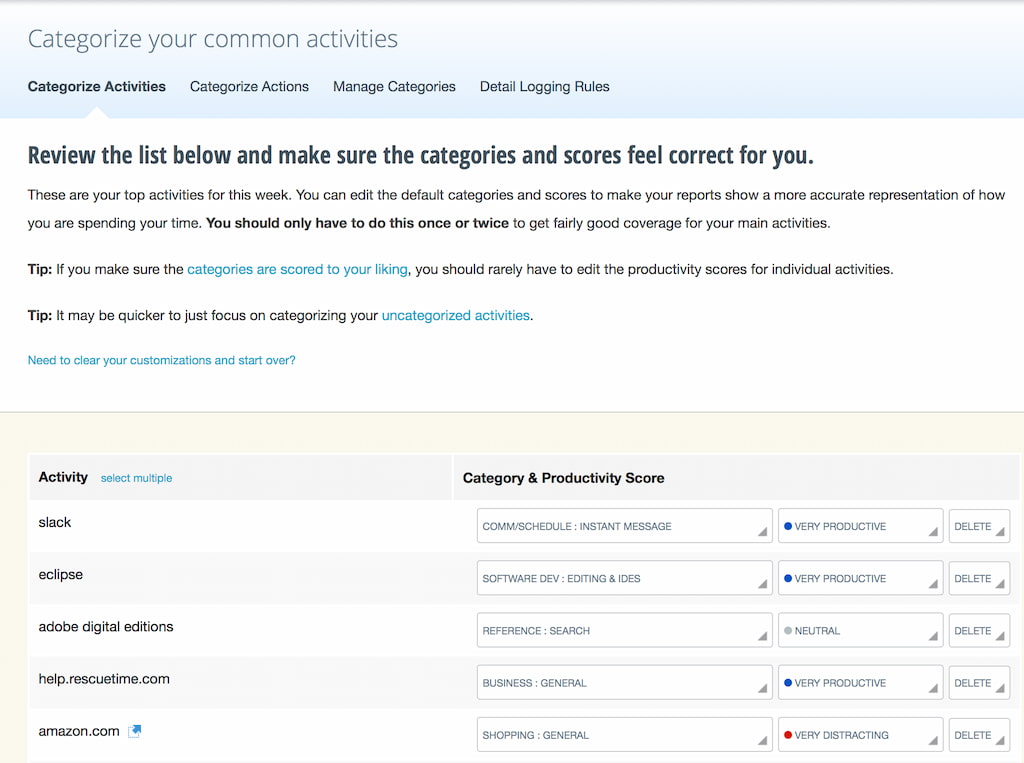Sure, here's a cleaned-up and detailed caption for the described image:

---

A screenshot from a website interface displays a section titled "Categorize Your Common Activities." Below the main heading, options include "Categorize Activities," "Categorize Actions," "Manage Categories," and "Detail Logging Rules." The introductory text advises users to review a list of activities and ensure the categories and scores accurately reflect their time usage for the week. It emphasizes that users can edit default categories and scores to get a precise representation of their productivity, suggesting that this adjustment process only needs to be done once or twice for comprehensive coverage.

Tips provided include the benefit of appropriately scoring categories to minimize the need for frequent edits and the efficiency of focusing on uncategorized activities. A prominent blue link offers the option to "Need to clear your customizations and start over."

Below this instructional text, a table is displayed with columns for "Activity," "Category," and "Productivity Score," listing various activities the user has engaged in.